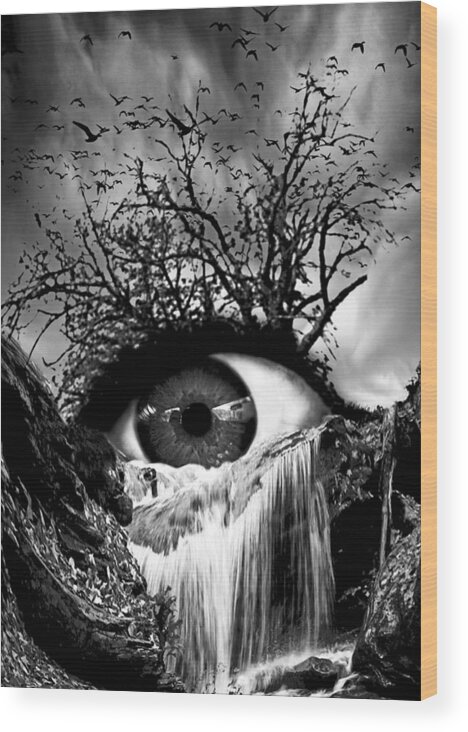This black and white image presents a surreal, horror-style scene dominated by a colossal, gaping human eye centrally located. The eye, set against a dark, gritty sky, has its upper lid seamlessly transforming into a tangled mass of tree roots or perhaps leafless, dead trees. From these roots, numerous ominous birds and possibly bats are eerily flying, filling the gloomy sky. Below the eye, resembling tears, a gushing waterfall pours forth, cascading down into a rocky valley, creating a powerful sense of a cosmic horror unfolding. The surrounding landscape consists of steep, sloped hills and a rugged, mountainous valley into which this torrent of water flows, magnifying the unsettling atmosphere of this intricate and bleakly mesmerizing scene.